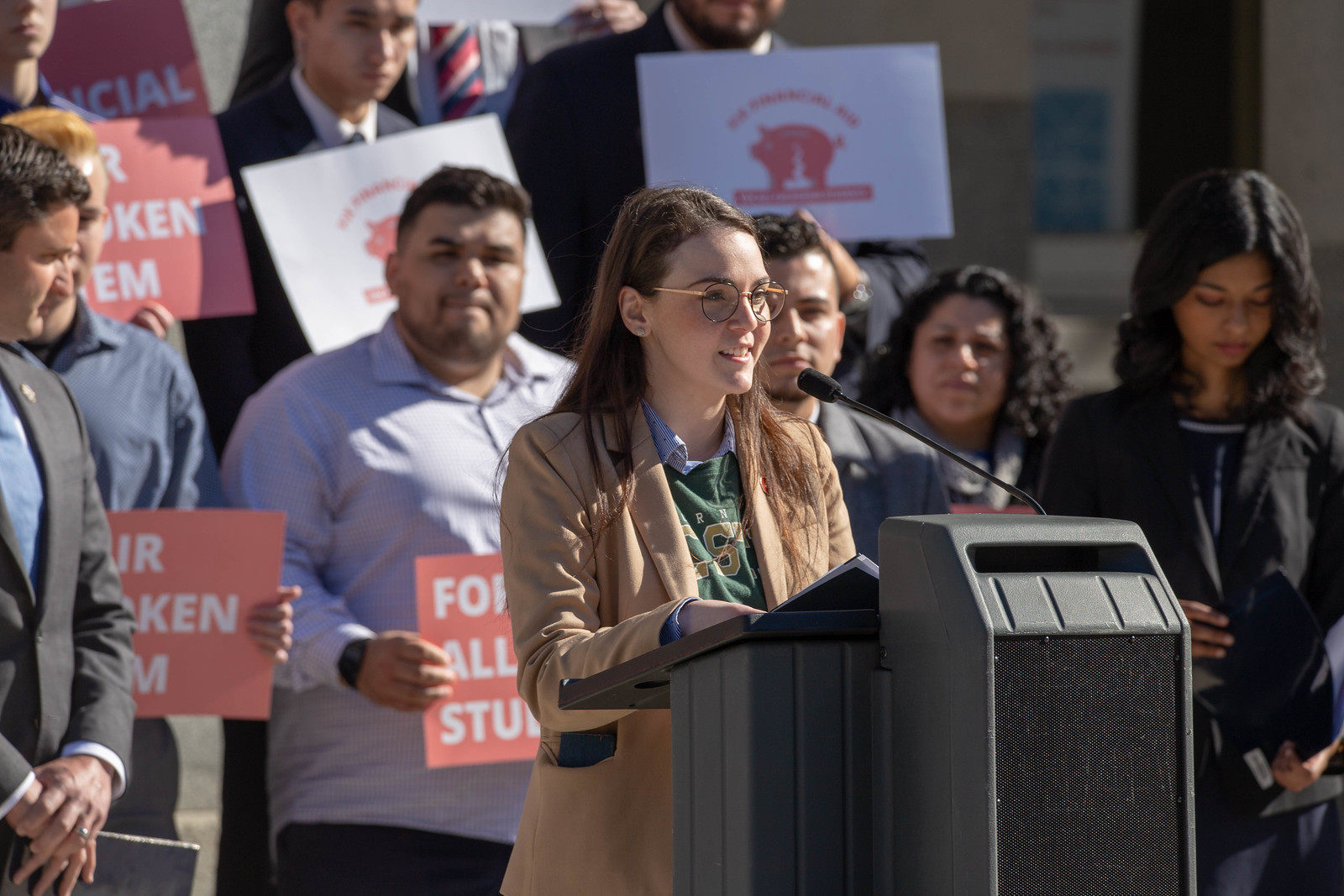In an outdoor setting, a young woman with straight brown hair and glasses stands at a black podium, making a speech. She's wearing a tan blazer jacket over a green shirt and appears to be gripping a notebook or book on the podium. The scene is set in bright daylight, with the sun illuminating the speaker. She speaks into a small black microphone, her focused demeanor drawing the attention of a diverse crowd behind her.

The backdrop consists of about eight people of various ages and ethnicities, all holding signs in support of her cause. The signs, which alternate between pink with white lettering and white with pink lettering, are partially obscured but suggest a protest or advocacy event. The group includes men and women, one of whom, positioned directly to her right (left side of the image), looks back at the crowd with folded hands. Among the signs, one appears to have a two-dimensional picture of a pig on it, indicating a possibly specific protest theme.

While most of the background figures are blurry, enhancing the focus on the woman speaking, they clearly create a scenic tableau of unified support and attention towards her impassioned speech.